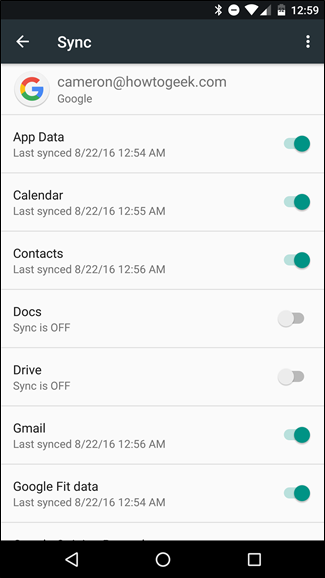This image is a detailed screenshot of a cellphone interface displaying sync settings for a Google account. At the top of the screen, a status bar shows various icons: a Bluetooth symbol, a Do Not Disturb icon represented by a circle with a line through it, Wi-Fi signal strength, cell phone signal strength at about 50%, a battery meter at roughly 75%, and a digital clock reading 12:59. 

Below the status bar, a gray header contains a left-pointing arrow, the word "SYNC" in uppercase letters, and a menu icon with three vertical dots, all rendered in white text. 

The primary section of the screenshot features a white background with the Google logo at the top, followed by the account email "Cameron at HowToGeek.com," and the word "Google."

Underneath, a line item indicates "App Data," which is switched on, showing the last sync date and time as 8-22-16, 12:54 AM. Following this, several service categories are listed: Calendar, Contacts, Docs, Drive, Gmail, and Google Fit Data. The items currently enabled for sync are App Data, Calendar, Contacts, Gmail, and Google Fit Data.

At the bottom of the screen, navigation icons include a left-pointing arrow, a circle (commonly the home button), and a square (recent apps button).

This caption provides a comprehensive description of the various elements and layout shown in the cellphone screenshot.